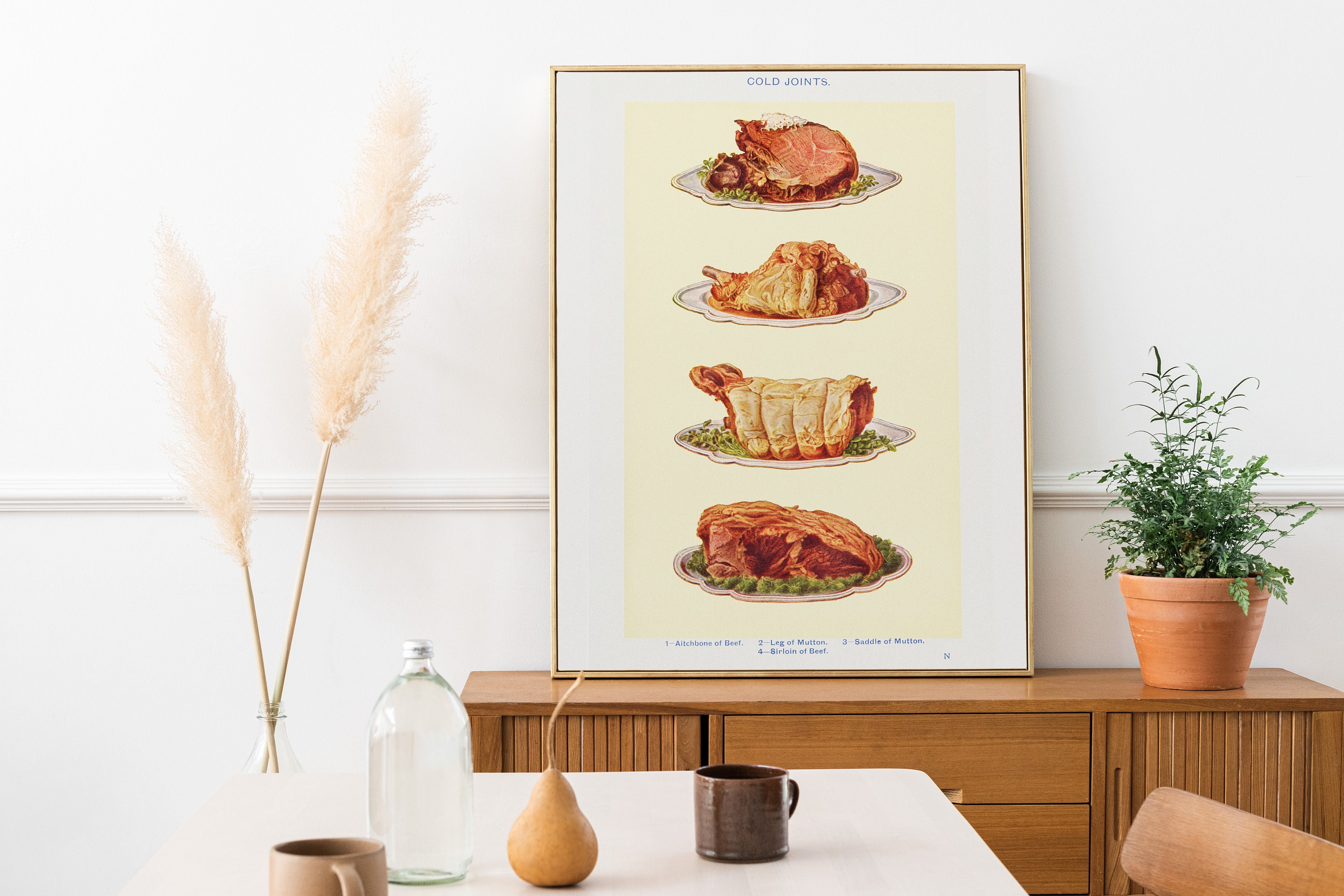In this detailed photograph of a kitchen scene, a brown wooden desk is positioned against a white wall in the background. On this desk sits a framed print illustrating various cuts of meat, including an H-bone of beef, leg of mutton, saddle of mutton, and sirloin of beef, each labeled in blue text beneath the images. To the viewer's right, there is a potted plant adding a touch of greenery to the setting. In front of this framed print, a white table spans the foreground, adorned with a centrally placed pear, an empty bottle to the left, and a brown coffee mug to the right. The entire composition captures a warm, rustic atmosphere, complete with a blend of white and brown hues, red and green accents from the plant, and tidy kitchen elements that enhance the inviting ambiance of the scene.